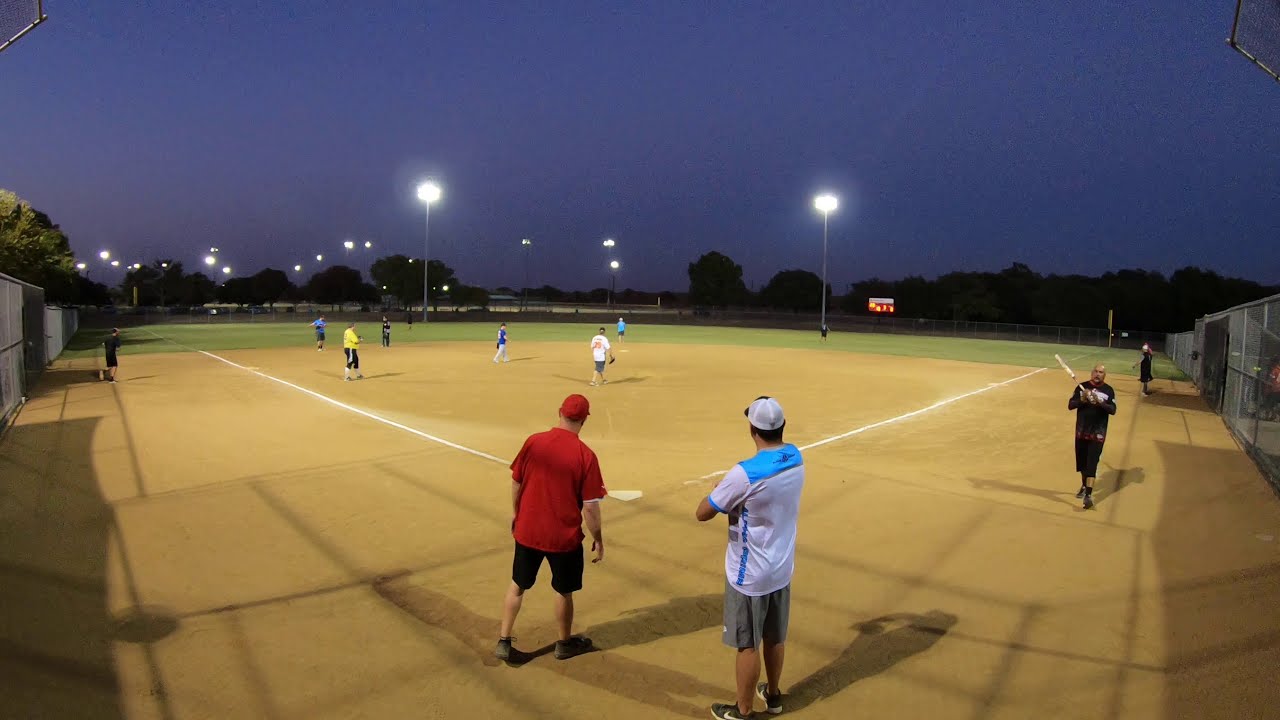The photograph captures a nighttime scene at a baseball diamond under illuminated skies transitioning to twilight, adorned with a purple hue. The field is clearly lit by several tall lights, casting bright beams over the light brown, muddy soil of the infield, which is marked by white-painted lines demarcating the bases. Surrounding the infield is a neatly maintained green grass outfield, with a silhouetted treeline forming the horizon. 

In the foreground, two men stand near home plate: one in a red t-shirt, black shorts, and a red cap, gazing towards the outfield, while beside him, another in gray shorts and a predominantly white shirt with blue accents, arms crossed and similarly focused on the field. To their right, a man in black shorts and a black shirt holds a bat, walking just shy of home plate. Surrounding them are several other individuals dispersed across the field, engaged in various activities, likely practice as no players are in position or running bases. None are wearing full uniforms, opting instead for casual sporty attire, further suggesting a practice session. A scoreboard is faintly visible in the distance, adding to the authenticity of the evening practice scene bordered by a protective fence.